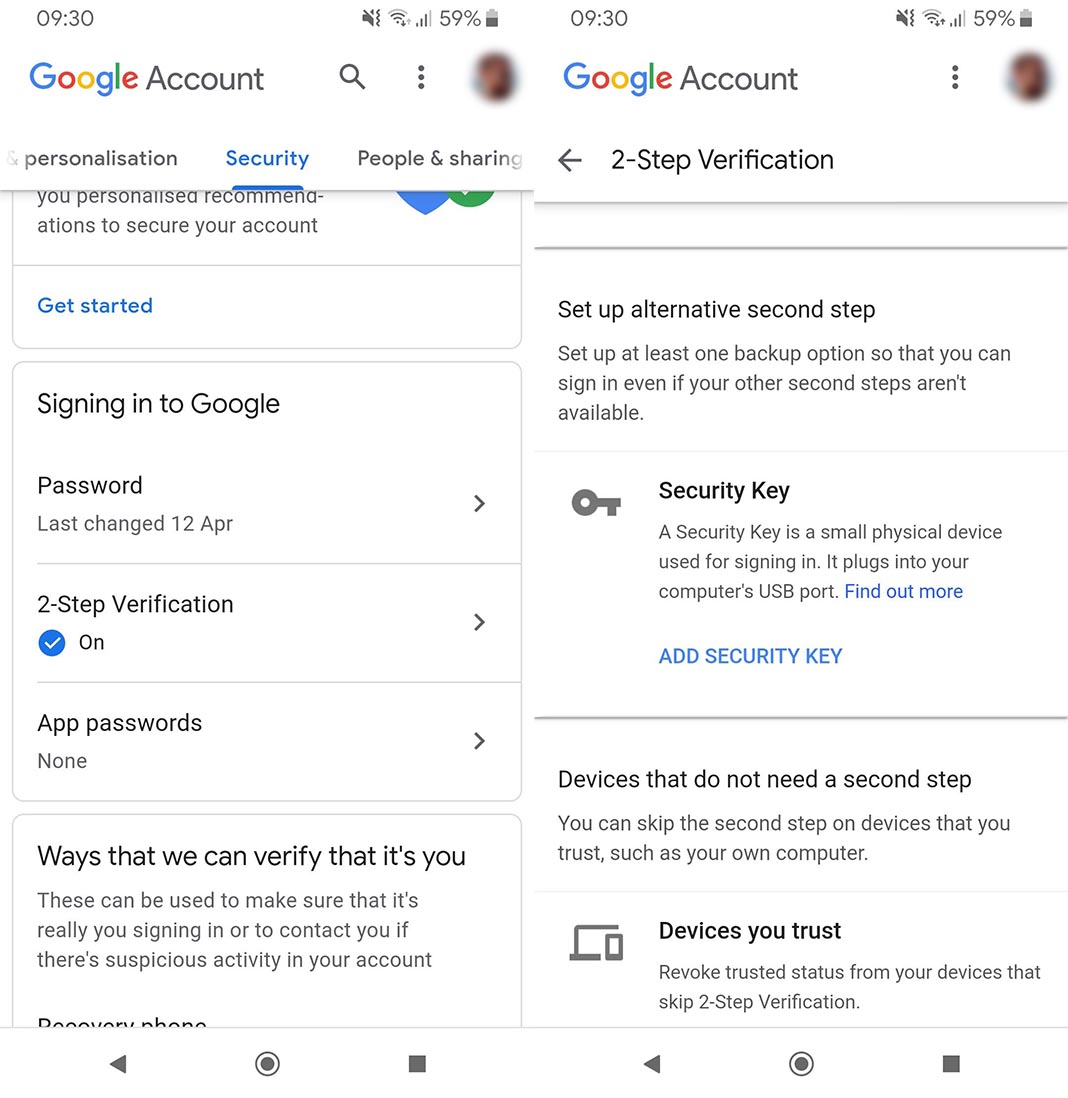**Caption:**
This image features two side-by-side screenshots from an Android phone, depicting various settings under a Google account. 

In the left screenshot, the top bar displays a Google logo in color, a search button, a three-dot menu icon, a blurred profile picture, and essential indicators including time, Wi-Fi signal, and battery status. Below this, the "Security" tab is selected, highlighted in blue. The main options listed include "Get Started," "Signing into Google," "Password," "Two-Step Verification," and "App Passwords," followed by sections like "Ways We Can Verify It's You." At the bottom of the screen, the standard Android navigation buttons are visible: a back arrow on the left, a home circle in the center, and a recent apps square on the right.

The right screenshot focuses on the "Two-Step Verification" screen. It includes a back arrow at the top-left corner, indicating the option to return to the previous screen. The screen presents options to "Set Up Alternate Second Step" and "Devices That Don't Need a Second Step," each accompanied by further informational content. This detailed setup allows users to enhance their account security efficiently.